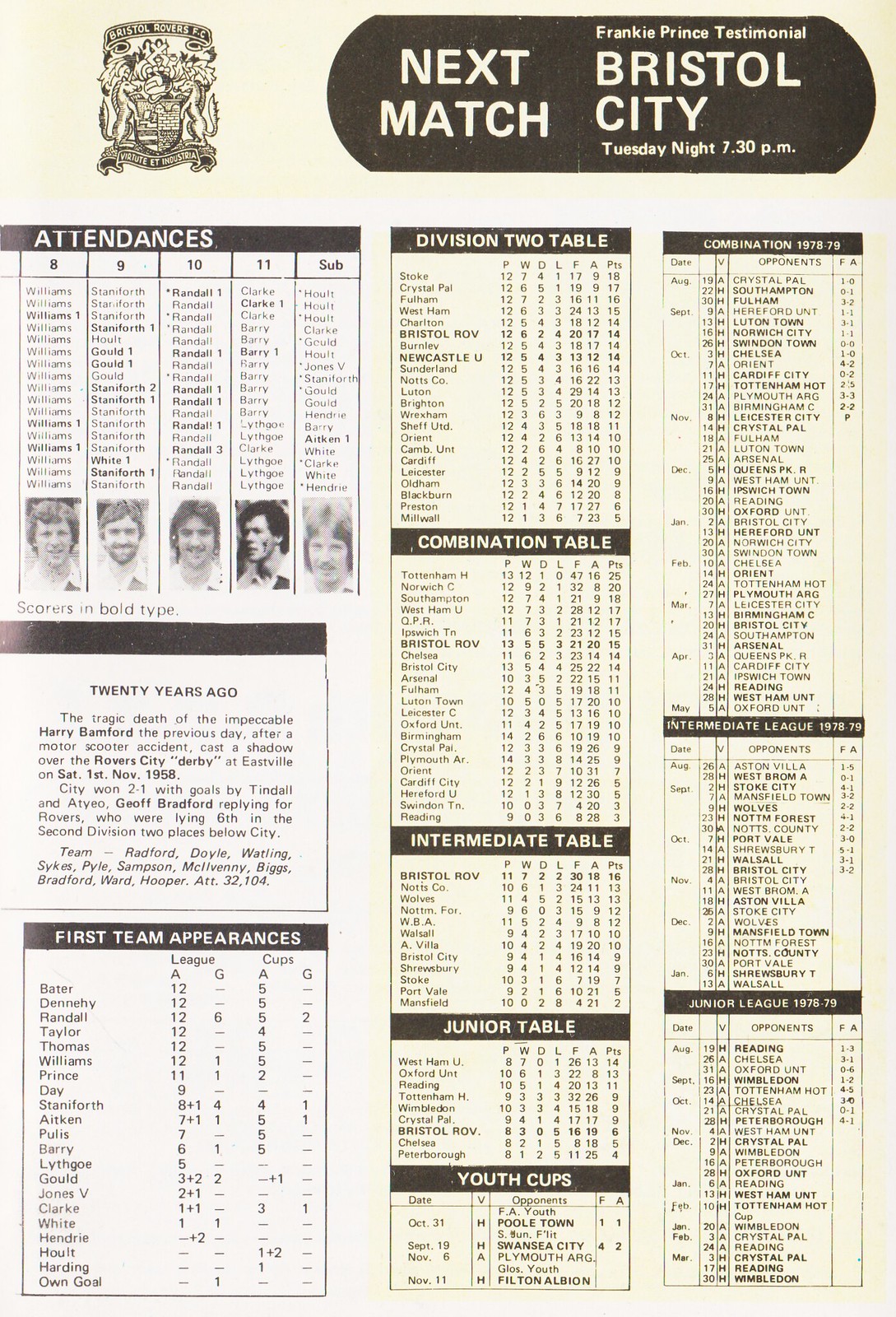This vertical rectangular image appears to be an aged program for an upcoming football (soccer) match, titled "Frankie Prince Testimonial," featuring Bristol City. The event is scheduled for Tuesday night at 7:30 PM. The program has a beige background covering the top and right side, displaying Bristol City's crest on the left side, alongside text indicating "Next Match: Bristol City" with further details on the date and time.

The right side of the program contains various statistical tables for the different divisions and categories such as the Division Two table, Combination table, Intermediate table, Junior table, Youth Cups, and leagues from 1978 to 1979. 

Additional features include individual player statistics under headings like "attendances" and "first team appearances." There are also five photos of young men, likely players, whose facial hair and style suggest the 1970s era. 

A memorial note is present, commemorating the 20th anniversary of the tragic death of Harry Branford, who passed away in a motor scooter accident on November 1st, 1958, right before the Rover City Derby at Eastville.